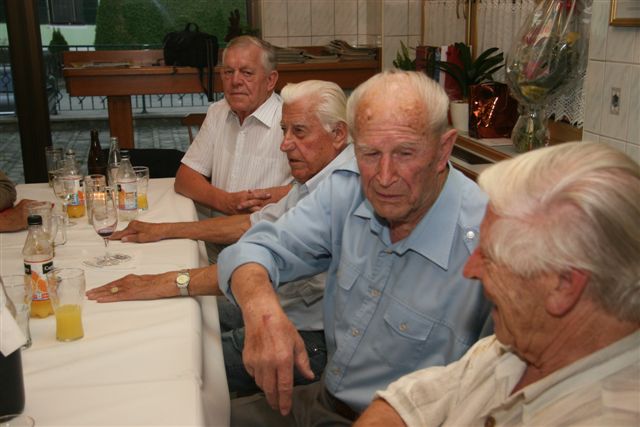The photograph captures a scene of four elderly men seated around a table adorned with a white tablecloth, located on the left side of the image. The table is laden with various bottles and glasses, some containing a yellow-colored liquid, possibly a fruit liquor cocktail, alongside wine bottles and glasses. The men appear to be engaged in conversation, though their expressions seem to reflect a sense of weariness or suffering. The man at the bottom right corner is dressed in a white shirt with white hair, the man next to him wears a blue shirt, followed by another man in a light-colored shirt, and finally, another man in a white shirt. In the background, there is a brown table with a black bag on it, and towards the top right, a bouquet of flowers can be seen. The setting resembles an old-fashioned diner or restaurant, evoking a sense of nostalgia and poignancy.